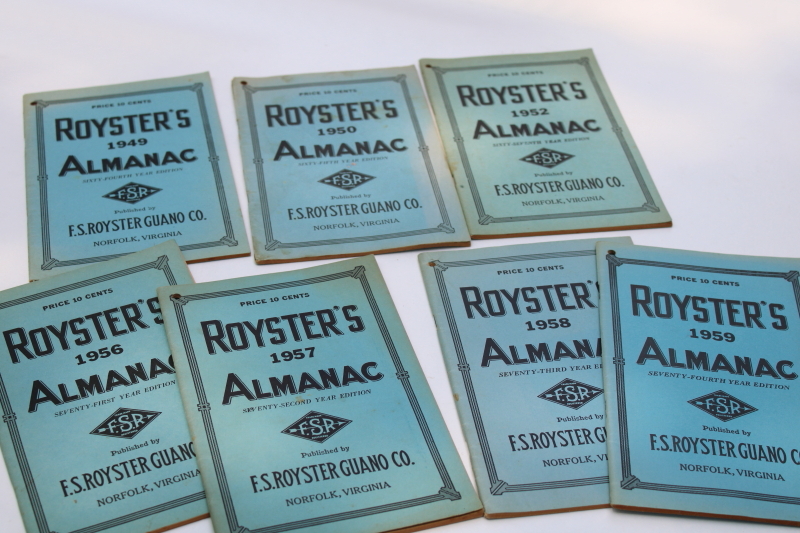This photograph showcases seven old almanacs titled "Royster's Almanac," spread out on a white table in two rows. Each booklet, primarily in shades of blue and bluish-teal due to varying degrees of fading, prominently features large black text within a rectangle border stating "Royster's Almanac," accompanied by a black diamond-shaped logo marked with "FSR." Beneath the logo, the publisher is identified as FS Royster Guano Company, Norfolk, Virginia. The almanacs, spanning the years from 1949 to 1959, show various levels of wear and coloration depending on their exposure, with dates clearly marking each edition. Specific annual editions noted include 1949, 1950, 1952, 1956, 1957, 1958, and 1959, with each year's edition number detailed on the cover.